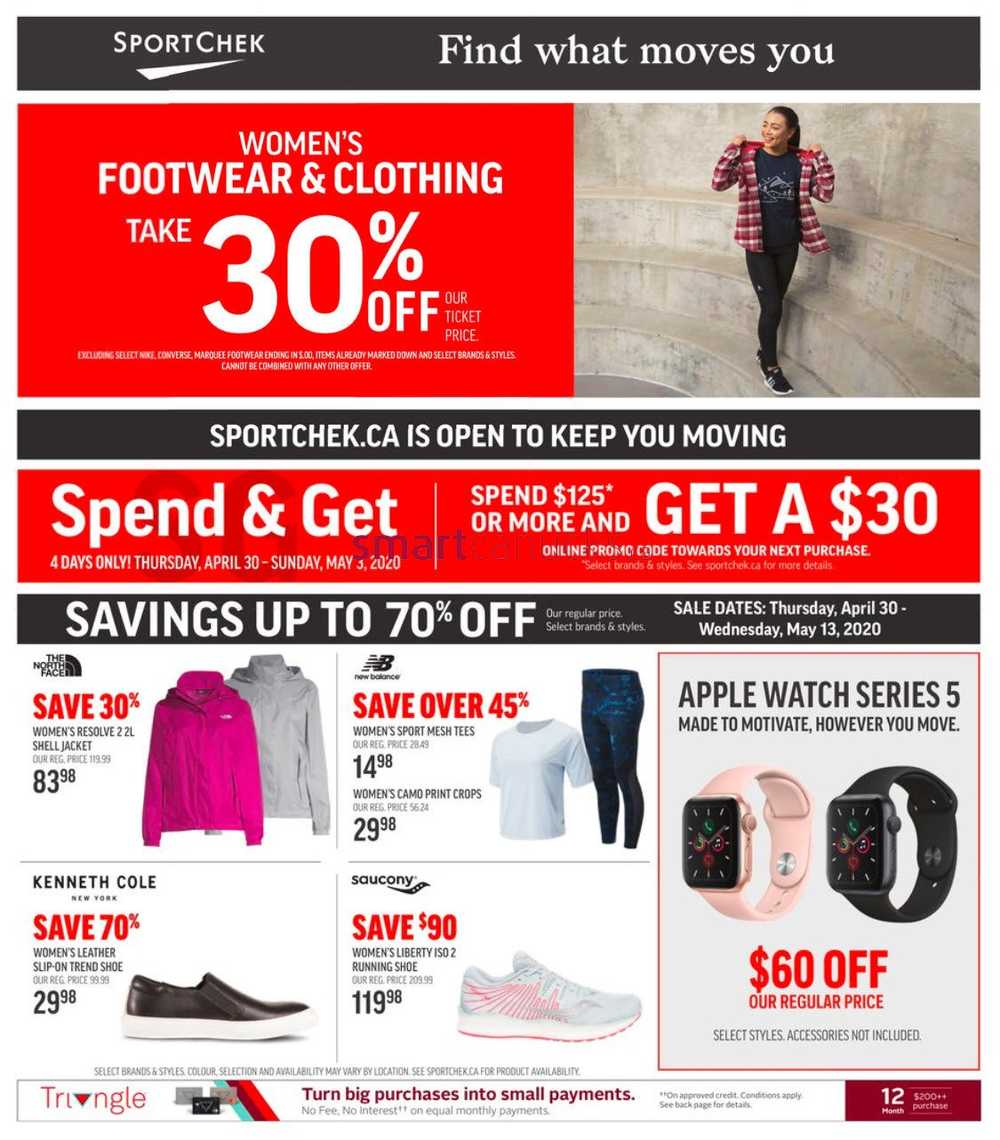At the top of the image, a dark gray header is positioned, featuring a slanted, white geometric shape resembling an arrowhead or triangle on the left side, with the text "Sport Chek" written in white beside it. To the right, a bold phrase "Find What Moves You," in a wide Times New Roman-like font, is displayed. 

Beneath this, a broad white strip runs horizontally across the image. Towards the left of this strip, a red banner announces "Women's Footwear and Clothing" with "Take 30% Off" written prominently in large white letters. At the bottom, on the right side of the red banner, small, hard-to-read disclaimer text appears in white.

To the right of the red banner, a woman stands on a stone walkway. She is wearing a plaid shirt, casually holding and popping the collar, with her head turned to the side. Her dark hair is tied back in a ponytail. She also wears a black graphic T-shirt and what look like black jeggings or leggings.

Further down, a black rectangle bordered by white areas on the top and bottom contains the text "SportChek.ca is Open to Keep You Moving" in white. Below this, another red banner, approximately three times the size of the previous black rectangle, reads "Spend and Get" in bold white letters. Underneath, smaller white text notes the offer duration with "Four Days Only! Thursday, April 30th - Sunday, May 3rd, 2020."